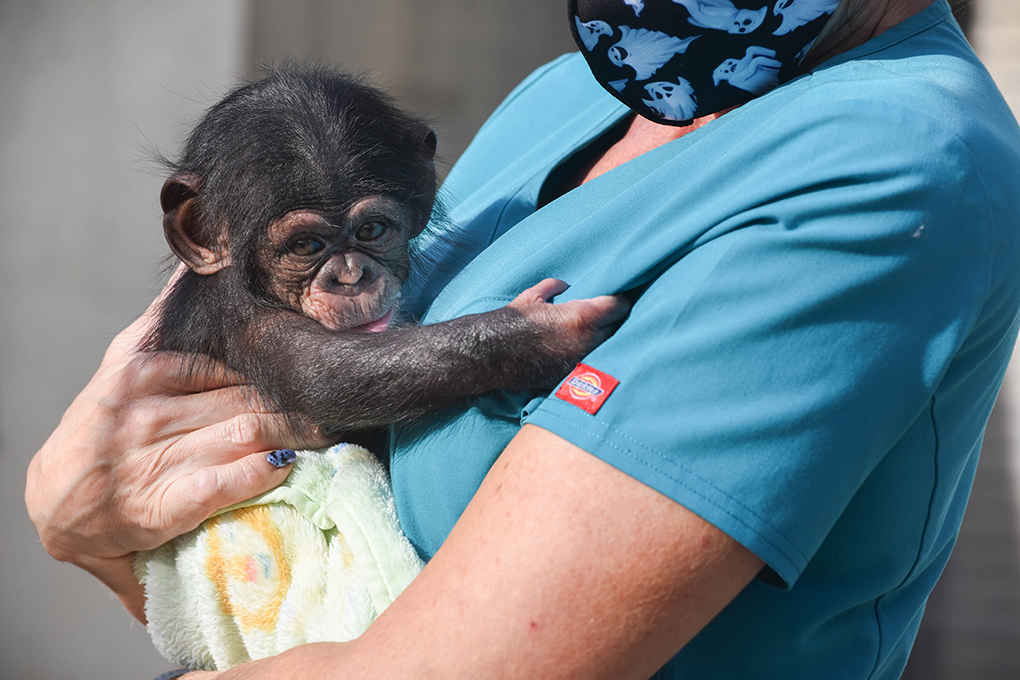In the foreground of this detailed color photograph, a female veterinarian is attentively holding a baby chimpanzee. Dressed in light blue Dickies scrubs with a distinguishable red and yellow tag, she also wears a black face mask adorned with blue and white ghost motifs, adding a touch of whimsy to her professional attire. The veterinarian’s fingernails are painted in a black and blue camouflage pattern, further illustrating her unique style.

Cuddled closely to her chest, the baby chimpanzee, with its black fur and lighter brown face, ears, and hands, clings to her for comfort and security. Its large dark brown eyes look inquisitively at the world around it. The veterinarian cradles the infant chimpanzee in a snug yellow blanket that features an orange-outlined lion with a red nose, adding a playful and warm touch to the scene. The chimpanzee, appearing very young—perhaps less than a couple of months old—holds on to the top of the woman’s scrubs as it nestles contentedly in the blanket.

The background is blurred, directing full attention to the touching interaction between the veterinarian and the baby chimpanzee. The side wall appears light gray, while the central area behind them features darker gray wood with lines, complemented by lighter gray shadows on the right side, creating a soft and subdued backdrop for this tender moment.